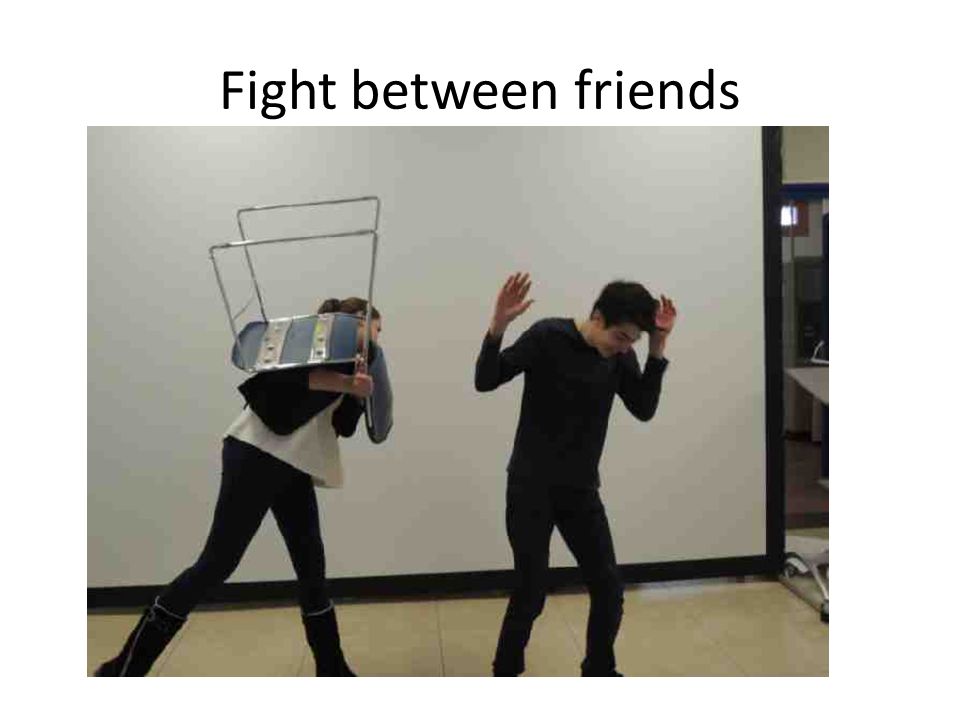The image, a still shot from what appears to be live footage or a movie, is of poor quality and captures a dynamic moment set against a large white backdrop with a black border. The floor is beige or tan tiles, and some furniture is visible in the background to the right. Above the scene, bold black text reads "Fight Between Friends," with the word "FIGHT" in uppercase and the rest in lowercase letters. The focal point of the photograph is two Caucasian individuals engaged in what looks like either play-fighting or enacting a scene. 

On the right, a man dressed entirely in black—wearing a long-sleeved shirt, pants, and shoes—has his arms up in a defensive stance, as if bracing for impact. On the left, a woman or girl is mid-action, raising a blue plastic student's chair with metal legs, appearing poised to throw or swing it at him. She is dressed in black boots, black pants, a white shirt, and a black vest or blazer. The scene suggests a staged or playful scenario rather than a serious conflict.